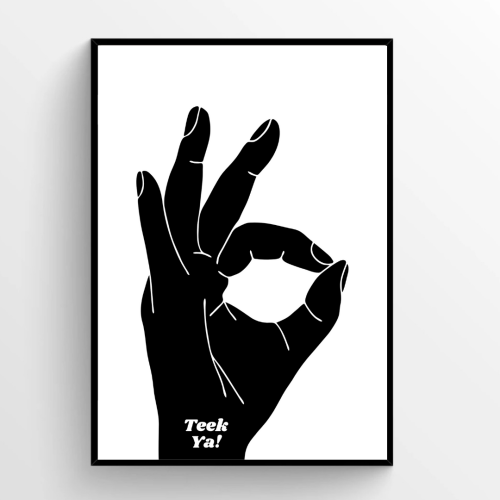The artwork features a black-framed, vertically oriented rectangular piece set against a light gray background. At its center, a white vertical rectangle with a black border showcases a black hand making an "OK" sign, where the thumb and index finger form a circle, and the middle, ring, and pinky fingers point upward. The black hand is detailed with white lines accentuating the creases and fingernails. At the base of the hand, the text "TIKYA!"—with "TIK" on one line and "YA!" on the line beneath—stands out in bold white capital letters. The hand's position and style, reminiscent of an "A-OK" gesture, imbues the artwork with dynamic character, blending both graphic design and symbolic hand language.